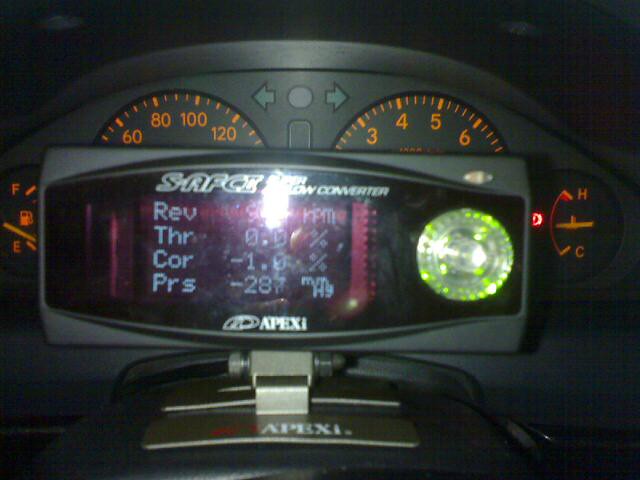This photograph captures the illuminated dashboard of a vehicle at night. The image is slightly wider than it is tall, providing a detailed view of the vehicle's interior from the driver's perspective. In the foreground, the top portions of two dials are visible, featuring orange lettering. The dial on the left displays numbers ranging from 60 to 120, indicating it is the speedometer. The dial on the right shows numbers from 3 to 6, corresponding to the vehicle's RPM gauge.

On the far right, the temperature gauge is centered with a red marker, and on the far left, the fuel gauge shows the needle hovering near 'E,' suggesting the vehicle is low on fuel. Dominating the center of the dashboard is a black electronic device attached to the steering wheel console, obstructing much of the instrumentation. This device features a green indicator light on the right side and a screen displaying "S-A-F-C-I-I" at the top, with reflective glare making it difficult to read the underlying text which appears to spell out "converter." Digital characters below this read "R-E-V-T-H-R-C-O-R-P-R-S," followed by numerical values and percent signs, the exact function of which is unclear.

Despite the night setting, the dashboard glows with a combination of digital and analog elements, offering a glimpse into the vehicle's operational status and the technological overlay introduced by the mysterious electronic device.